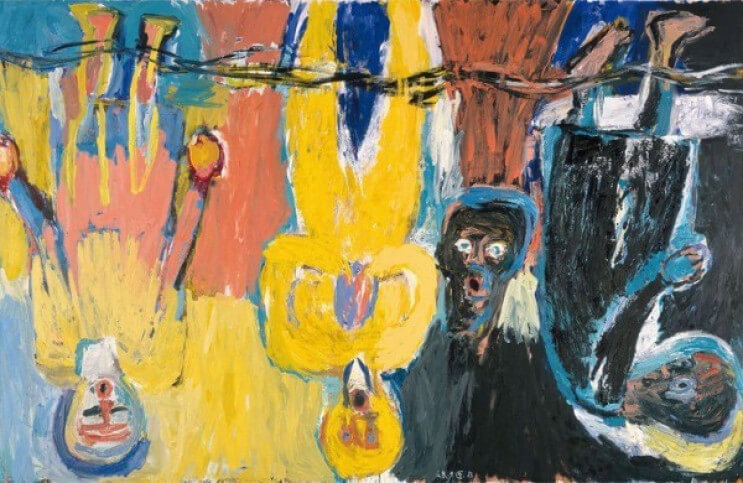The image is a vibrant painting featuring four human figures, with three suspended upside down and one in an upright position. The figures dangle from a wire-like string stretching from the left to the right side of the painting. The first figure on the far right is upside down, wearing black pants with a blue streak on its arm and a yellow detail on the back of its head. Its head is turned to the right, and it shows a stunned expression with an "O-face." The second figure, next to the first, is also upside down. Only its head is visible, displaying black facial tones, an open mouth, blue and black hair. The third figure from the right is fully yellow with hands positioned over its chest at a 90-degree angle, featuring a white neck and an open mouth. The fourth figure, on the left, is right-side up, adorned in multi-colored attire: pink and blue pants with blue at the bottom, potentially pink boots or shoes, and a yellow top. It has blue hair, red lines on the forehead, visible eyebrows, an open mouth, and a red nose. The entire composition utilizes solid primary colors like yellow, blue, pink, black, white, an off-shade green, and gray. Each figure exhibits a wide-eyed, surprised expression.